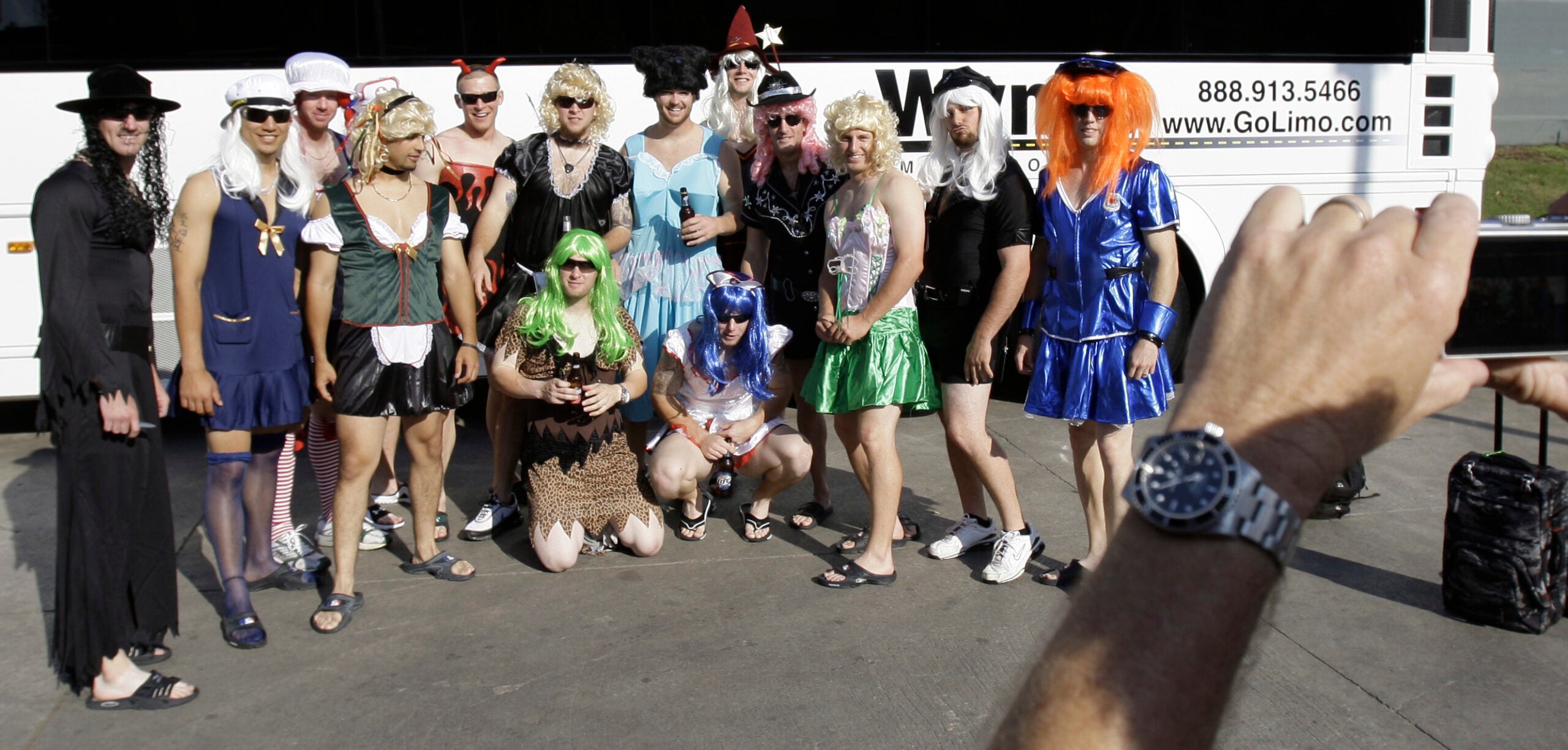The outdoor image captures a group of 16-17 men dressed in various drag outfits standing in front of a white travel bus that displays "www.golimo.com" and "888-913-5466." The men wear an assortment of colorful and whimsical wigs, ranging from bright orange and green to stark white, with some sporting outlandish accessories such as devil horns and wizard's helmets. Their costumes vary widely, including a shiny blue schoolgirl uniform, a sailor's outfit, and even a prehistoric getup. Despite the comedic and exaggerated nature of their appearance, suggesting it's a humorous event or performance rather than a serious attempt at crossdressing. In the foreground, a man wearing a wristwatch is visible, capturing the scene with his camera. The background includes a clear sky, some clouds, and grass, suggesting a sunny day.